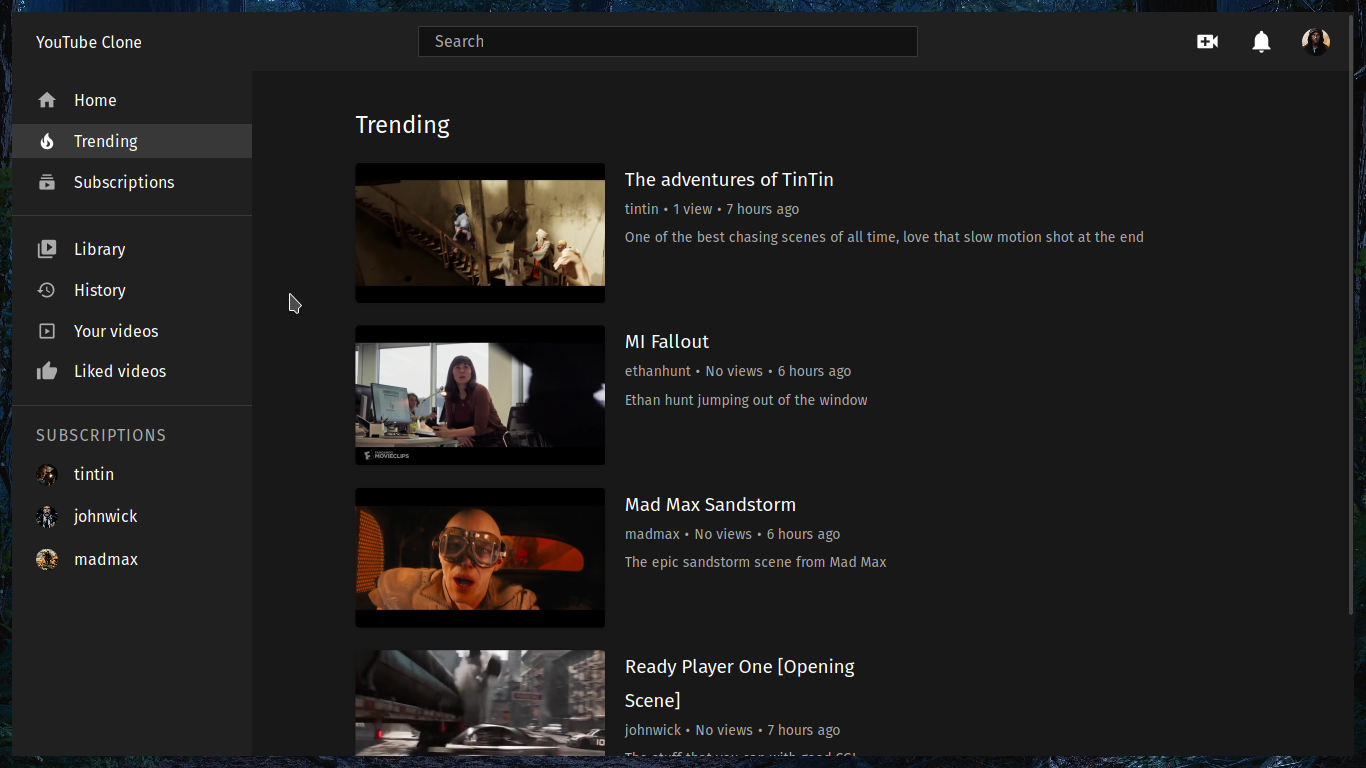In the image, we see a digital recreation of a YouTube interface, likely a YouTube clone. At the top right corner, a profile picture of an individual with dark skin, black hair, and wearing a black jacket is visible. Next to the profile picture, there is a bell icon for notifications and a video camera icon. 

Central at the top, a search bar is prominently placed, with the word "Search" in white text on its left side. On the top left, the title "YouTube clone" is displayed. Moving down from the top left, several navigation categories are listed: Home, Trending, Subscriptions, Library, History, Your videos, and Liked videos. Below these categories, under the Subscriptions section, three channels are named: Tintin, John Wick, and Mad Max.

The main content area showcases four video thumbnails in a grid. The top video is titled "The Adventures of Tintin," followed by "Am I Fallout" for the second video, "Mad Max Sandstorm" as the third, and "Ready Player One Opening Scene" as the last video at the bottom. Each video has a corresponding thumbnail image representing its content.